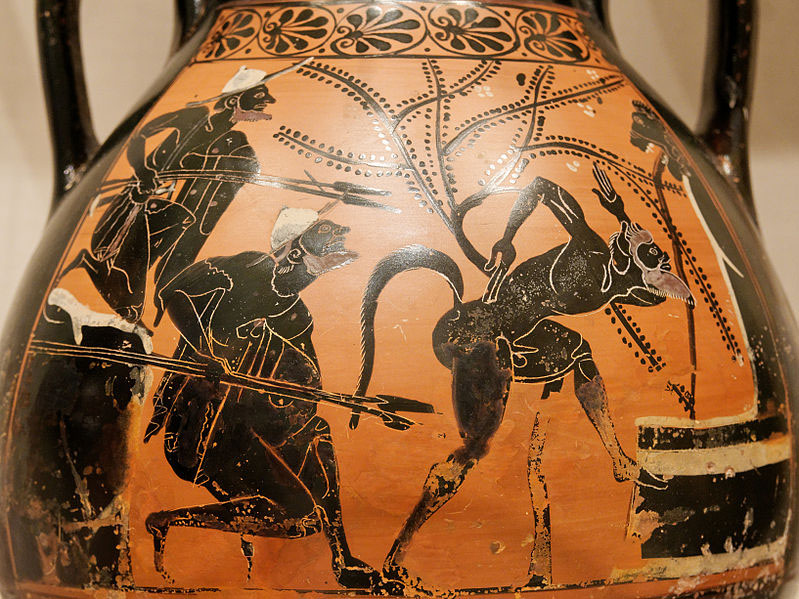This image depicts a close-up of an ancient vase, possibly originating from North Africa. The vase's background is light brown, adorned with intricate, darker brown designs. It features two slender, black handles on either side and has a bulbous middle with a skinny neck and an orange panel near the top. The upper section is decorated with a rectangular band of sideways flowers, each alternating in orientation and extending from curved lines.

Central to the vase's artwork are three humanoid figures. The leftmost figure, perched on a rock, holds two spears and wears what appears to be a white cap. The middle figure, slightly larger, mirrors the first but stands on the ground. The third figure resembles a goat-man with a tail and appears to be walking. To the right, partially cut off in the image, is a lion-headed figure with a walking stick. The scene suggests a hunting narrative, emphasized by the hunters and their prey. The vase's surface shows signs of age, being faded and scratched, enhancing its ancient and museum-worthy appeal.